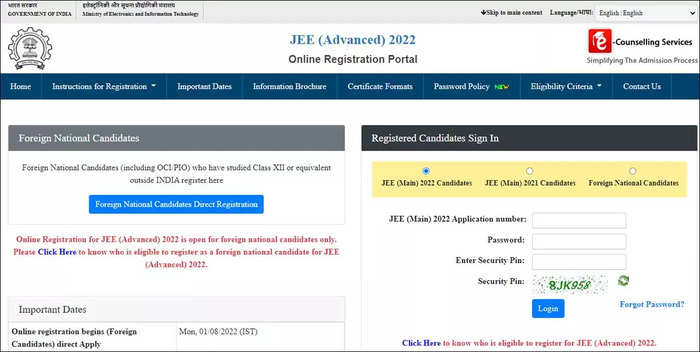The image depicts a semi-blurry screenshot of the JEE Advanced 2020 online registration portal, with layout elements and text partially obscured. The webpage appears to be an advanced registration platform, potentially catering specifically to candidates, including foreign nationals, for the JEE Advanced 2020 counseling services.

At the top of the page, a series of navigation buttons link to important sections such as Home, Instructions for Registration, Important Dates, and an Information Brochure. Below this navigation bar, there's a section designated for foreign national candidates featuring a prominent blue button labeled "Registration for Candidates."

A bold red notice beneath this section emphasizes that online registration is for foreign national candidates only. Important registration dates are noted, including a specific date, Monday, 1-8-2022. On the right-hand side, a separate section enables registered candidates to sign in, accommodating candidates from both JEE Main 2022 and 2021, as well as foreign national candidates.

This sign-in area includes several input fields: one for the JEE Main 2022 application number, another for the password, and a third for a security pin (likely akin to a CAPTCHA for verification purposes). A blue login button is positioned directly below these input fields for user authentication.